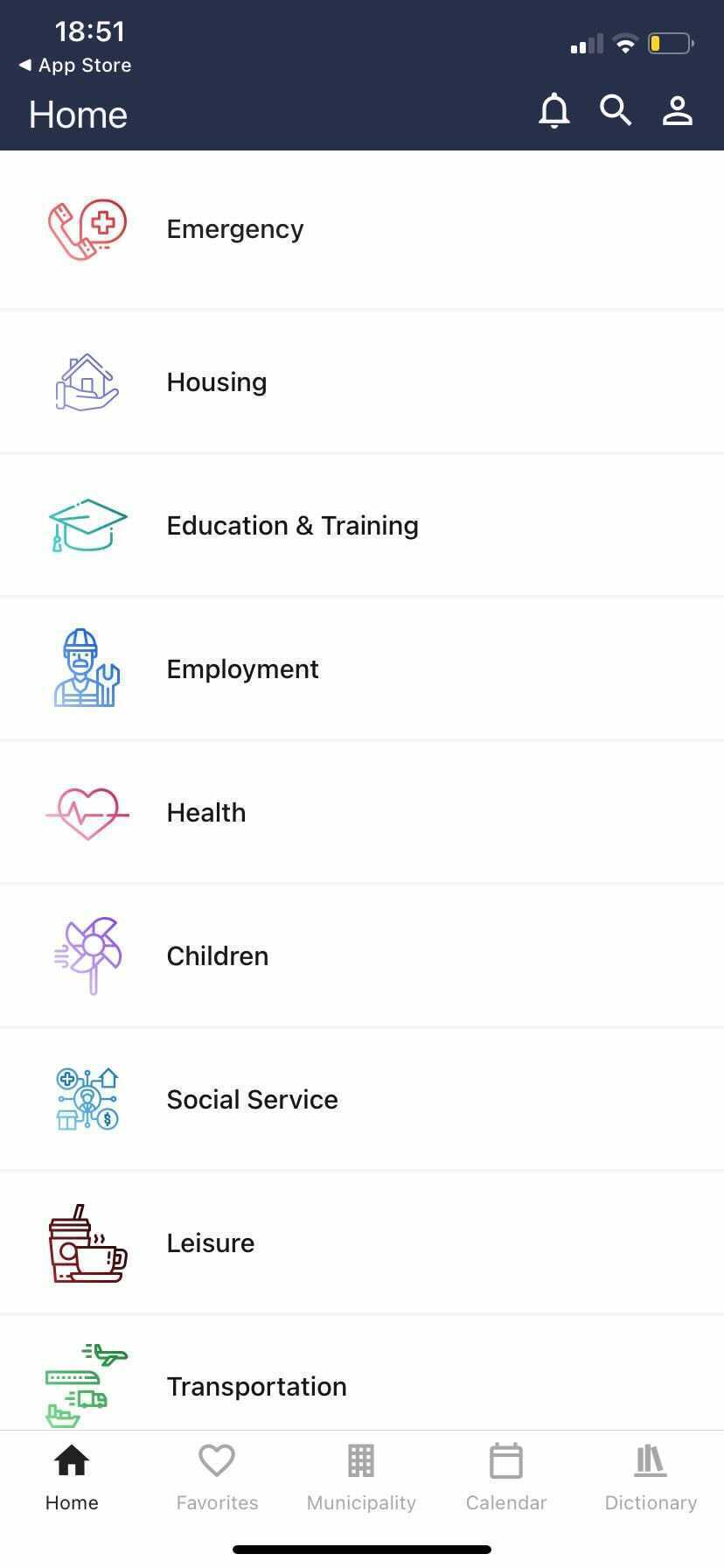The image is a screenshot taken from a cell phone, depicting a detailed user interface. At the top, there is a black header with white text. In the upper left corner, the time is displayed as 18:51. Directly beneath this, there are textual labels that read "App Store" and "Home." In the upper right corner, there are status icons showing two out of four signal bars, an active Wi-Fi connection, a low battery indicator, a notification bell, a magnifying glass, and an icon representing a person.

The main content is set against a white background and consists of a vertical list of categories, each accompanied by a relevant icon. The categories, read from the top, are as follows:

1. **Emergency**
2. **Housing**
3. **Education and Training** - Illustrated with a green-outlined graduation cap.
4. **Employment**
5. **Health** - Represented by a red heart icon.
6. **Children** - Marked with a purple pinwheel icon to the left.
7. **Social Service**
8. **Leisure** - Depicted by a cup of coffee icon.
9. **Transportation** - Accompanied by icons representing an airplane, a train, a boat, and a truck.

This detailed layout suggests that the provided screenshot may be from an application or service directory that helps users navigate various essential categories and services.